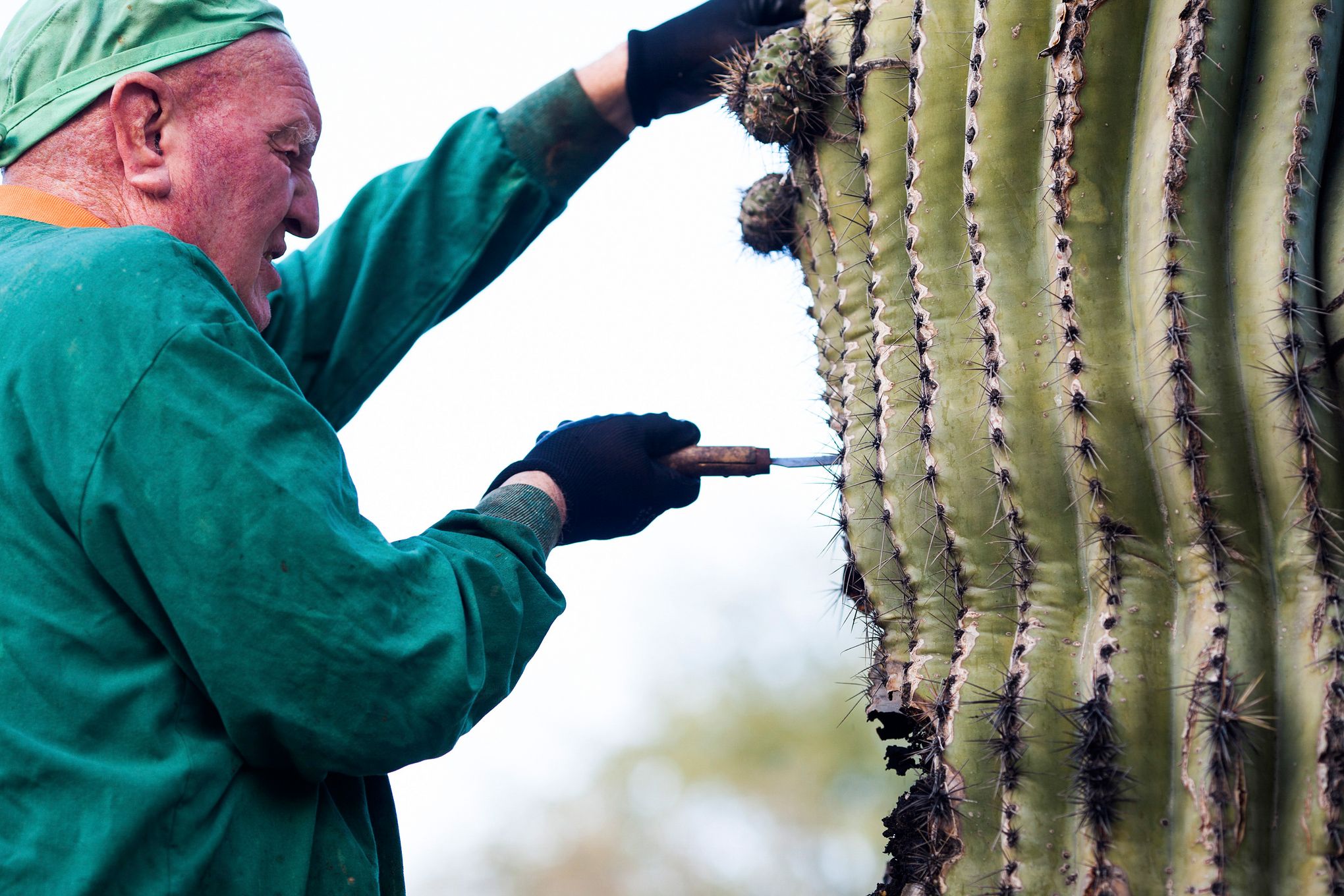The photograph captures an older man engaged in the delicate task of tapping into a massive cactus. Positioned on the left side of the image, the man wears attire resembling medical scrubs or a surgeon's outfit, suggesting a layer of protection. His ensemble includes a linen cap, a long-sleeve green shirt, and gloves, presumably safeguarding him from the cactus's formidable spines.

With a tool in hand—a wooden-handled instrument with a metal edge—the man meticulously works on the cactus, which towers with the girth of a large tree trunk and features menacing black spikes. Despite the apparent danger posed by the cactus's numerous sharp spines, the man appears focused and intent on extracting something from within the plant.